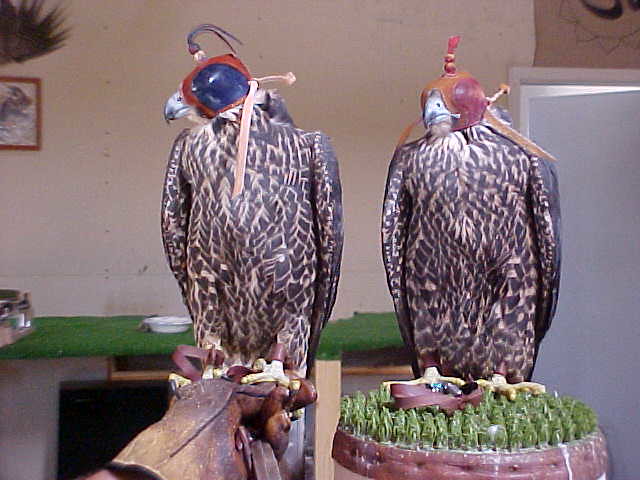This color photograph, captured in landscape orientation, depicts two ornately crafted figural birds, which appear life-sized and realistic but are actually artificial. The birds, which are often mistaken for owls or falcons, are perched side by side in a crafted tableau. The bird on the left is perched on a block of wood with what seems to be a rubber band or a decorative head covering—possibly a hood—on its head; the head is adorned with red and orange details and a blue circle around the eye, and it faces left in profile with a beige strap around its neck. The bird on the right, perched on a stump adorned with greenery, sports a similar hood with red covering its eyes and an ornamental plume on top. The birds have white beaks and their eyes are either closed or made to appear closed, possibly through photo editing. Behind them stands a beige wall adorned with a bowl, fake grass, shelves, and wall plaques. The overall photographic style leans towards representational realism, capturing every detail meticulously despite the clarity issues noted.